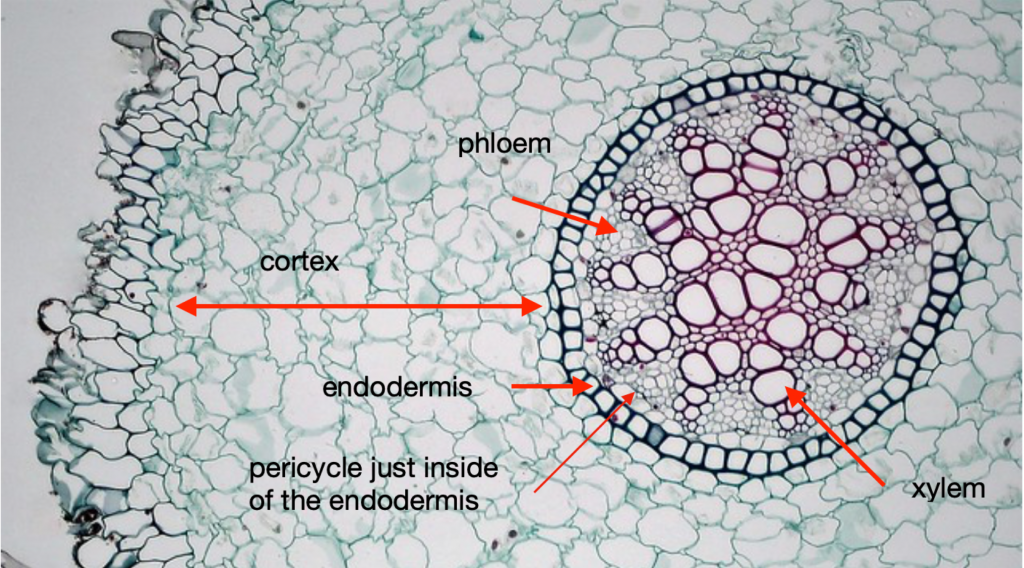This image is a detailed scientific diagram of a multicellular structure, featuring vibrant colors and intricate labeling. Central to the image is a circular core, where the xylem is located, distinguished by a purple hue. Surrounding this core is the endodermis, outlined in dark green, with the pericycle just inside of it. The cortex encompasses this region, highlighted by shades of green and blue. The phloem is also labeled within the inner structure. Red arrows and text annotations point to each of these features, including the cortex, endodermis, pericycle, xylem, and phloem. The background of the image appears to be a light gray. The combination of colors and detailed labeling lends a kaleidoscopic and educational quality to the depiction, making it a visually striking representation of cellular anatomy.